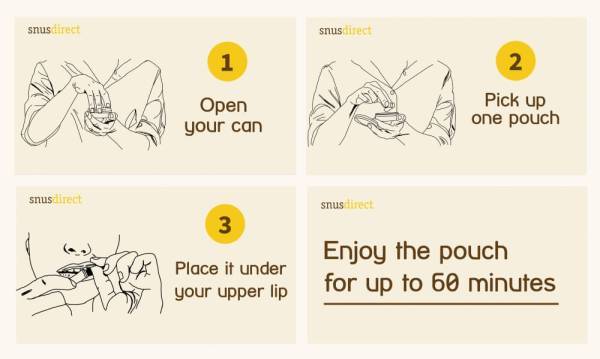This detailed caption provides an in-depth description of a diagram designed to guide the user through a process. The image has an off-white background and is rectangular in shape, oriented in a landscape view. At the top left corner of the rectangle, the word "SNUS Direct" is prominently displayed. The rectangle is divided into four quadrants, each providing a sequential step in the process.

**Upper Left Quadrant: Step 1**
- Instruction: "Open your can"
- Accompanied by a black-and-white illustration demonstrating the act of opening a can.

**Upper Right Quadrant: Step 2**
- Instruction: "Pick up one pouch"
- Features a black-and-white drawing showing the selection of a single pouch from the opened container.

**Bottom Left Quadrant: Step 3**
- Instruction: "Place it under your upper lip"
- Illustrated with a black-and-white diagram highlighting the placement of the pouch in the user's mouth, specifically under the upper lip.

**Bottom Right Quadrant: Step 4**
- Instruction: "Enjoy the pouch for up to 60 minutes"
- This quadrant does not include an illustration, focusing solely on the text.

The text throughout the diagram is presented in a dark brown font, while the instructional drawings in the first three quadrants are rendered in black and white, providing clear visual guidance alongside the text.